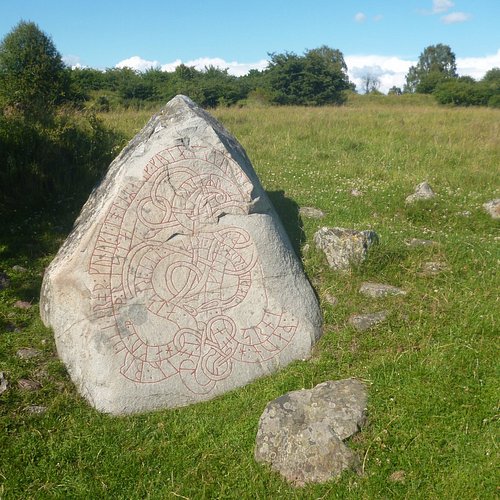The image captures a green grass field scattered with various boulders and rocks firmly embedded in the ground. Central to the composition is a prominent rock that presents an intriguing sight with its etched, serpentine patterns and intricate red markings, suggesting a complex design that intertwines like yarn. Certain sections of the etchings appear to depict ambiguous letters, including possible identifiers like 'I', 'R', 'P', 'H', 'A', and 'F'. The rock itself seems roughly triangular at the top, tapering down to a more rounded base. Behind this focal boulder, the landscape features a plethora of green-leafed trees that stretch to the horizon, and upon closer inspection, fluffy trees can be noticed to the far left. Above, a tranquil blue sky dotted with puffy white clouds enhances the serene daytime setting, with sunlight bathing the scene.